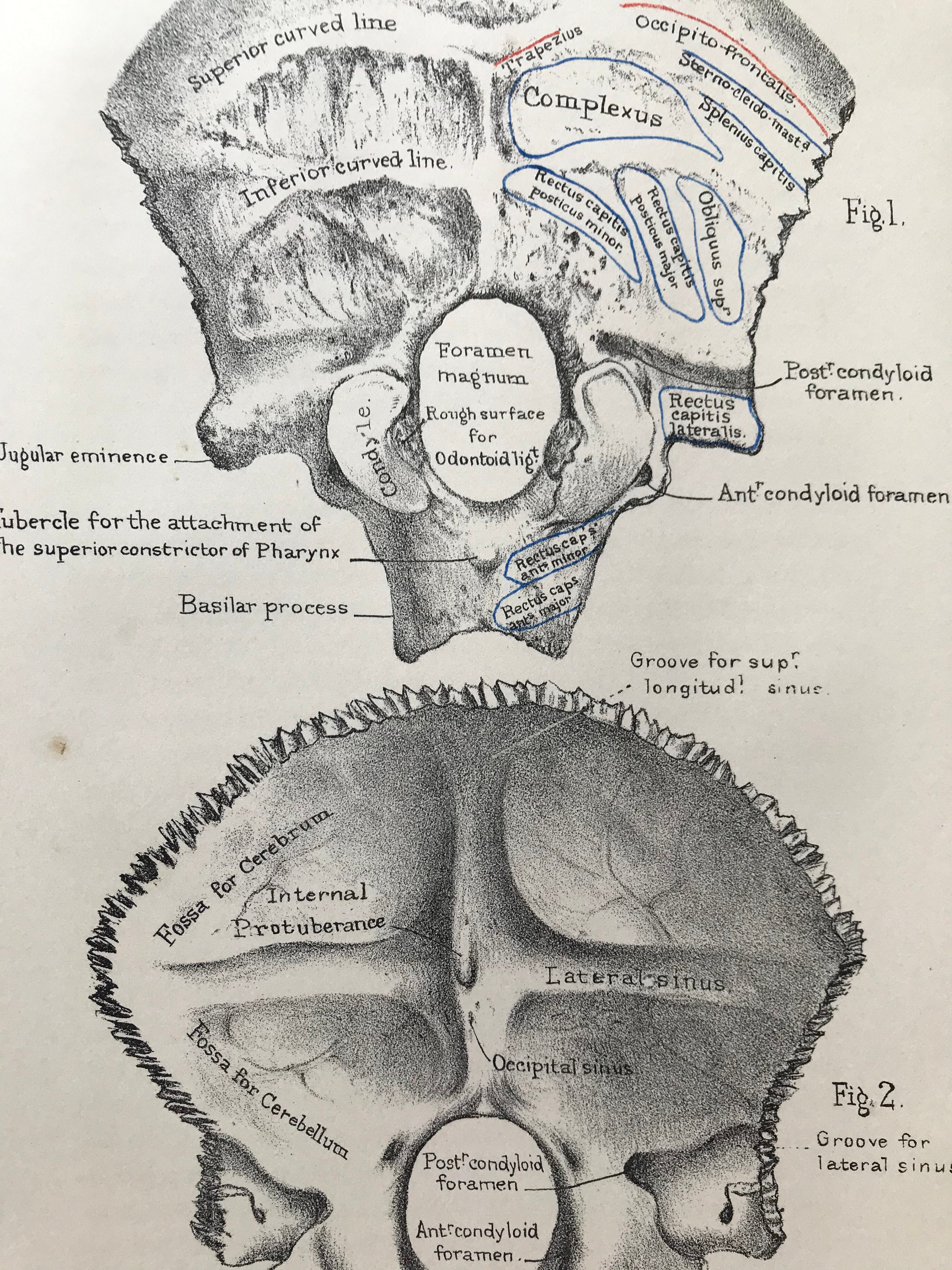The image features black and white, pen and ink scientific illustrations of a human skull, showcasing two figures with detailed anatomical labeling. Figure One, positioned at the top, displays a frontal view of the skull, marking various parts such as the superior curved line, occipital frontalis, trapezius, complexus, and jugular eminence. Figure Two at the bottom presents a top view of the skull, illustrating components like the fossa for cerebrum, lateral sinus, fossa for cerebellum, post-condyloid foramen, and groove for lateral sinus. The labels, written in a foreign language, denote intricate structural details, suggesting the diagrams are likely sourced from an old anatomy textbook or medical reference guide.